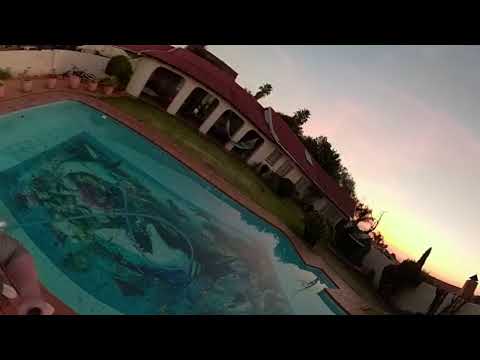This image captures the backyard of a house featuring an in-ground pool needing cleaning. Surrounding the pool, there are various potted plants in orange containers, as well as green bushes and trees. The pool deck is made of orangish bricks, and the pool itself displays a vivid blue with a painting of blue and white sharks showing their sharp teeth at the bottom. 

The house, which is white with a red roof, is bordered by a white fence dividing it from a neighboring house with a similar roof. In the distance, there is a grill and more greenery, while the sky above shows a mix of blue and grayish clouds and a hint of yellow, indicating sunset. The image is slightly blurry, with a finger visible at the bottom left corner and a black line stretching across the top and bottom.